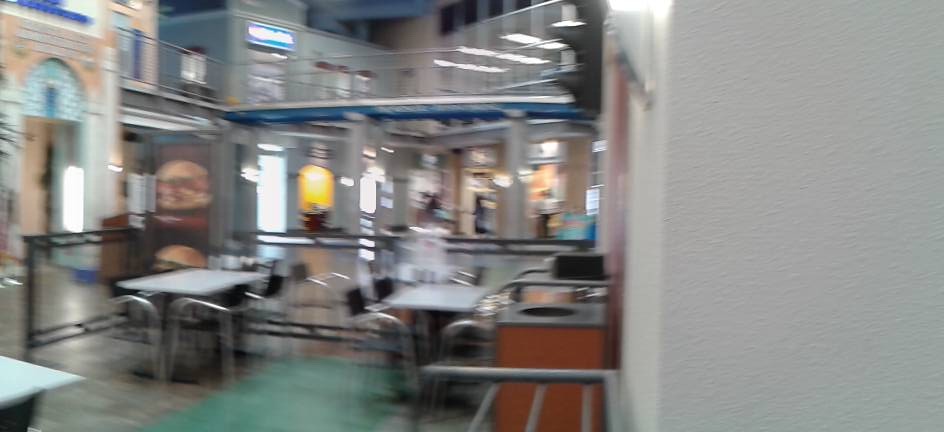A blurry, out-of-focus color photograph capturing a bustling indoor scene, likely inside a shopping mall. The image is in landscape orientation, featuring a gray wall prominently on the right-hand side. In the foreground, two sleek gray tables are accompanied by chrome chairs with low black backs, arranged neatly. Adjacent to the wall on the right is a dark brown trash can with a flat black lid, marked by an open slot. The setting appears to be a food court area on the ground floor, with the second level visible above. Neon signs punctuate the upper level, hinting at various stores or eateries. The overall atmosphere is reflective of a busy, multi-story commercial space.